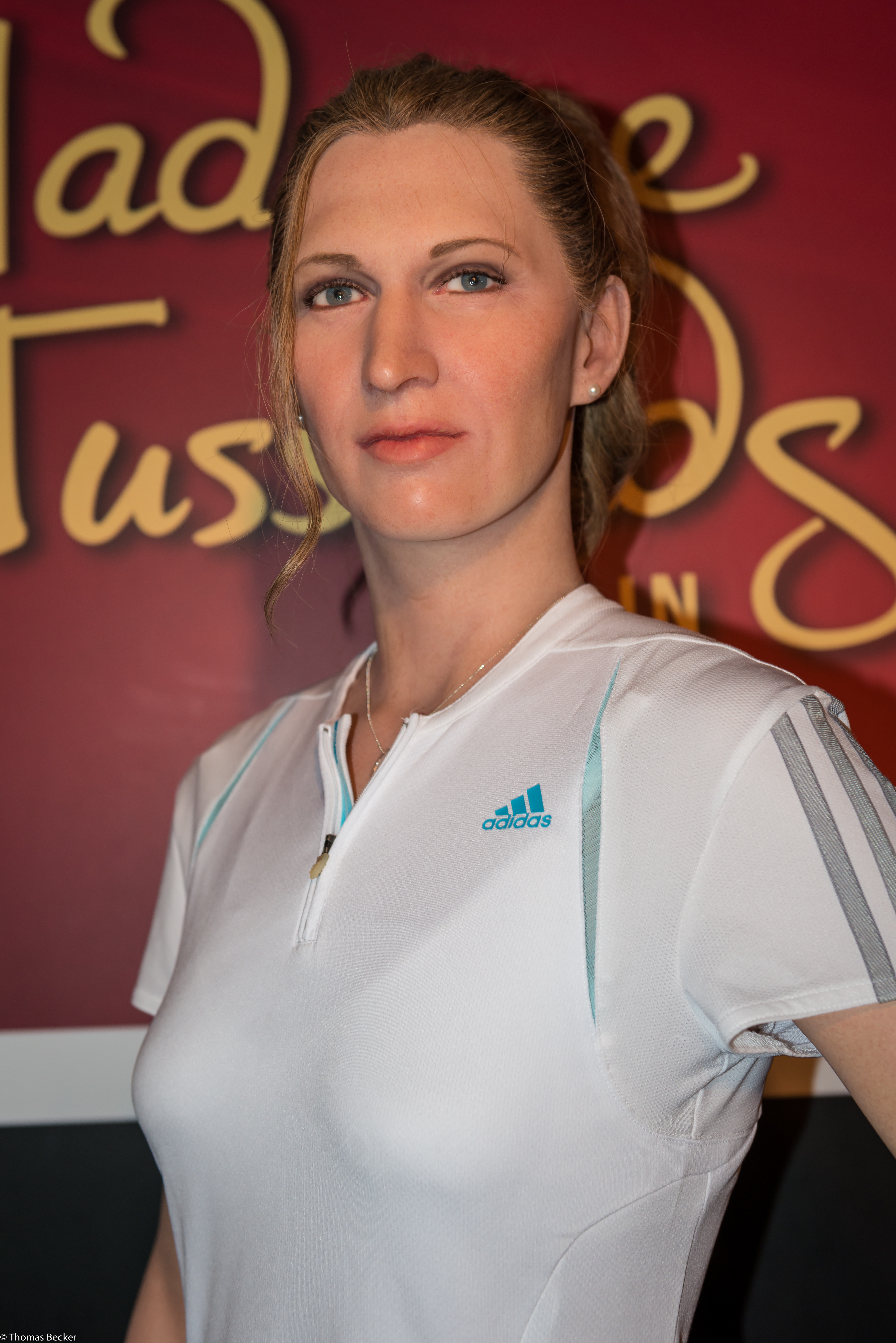This tall rectangular photograph captures a highly realistic wax museum figure of a woman, visible from the torso up, facing forward with a slight tilt to the left. She has pale skin, dark blonde hair, and light blue or gray eyes, wearing a serious expression. The woman is dressed in a white zip-up athletic t-shirt with gray stripes on the short sleeves, under which a white sports bra is visible. The t-shirt, featuring a prominently displayed teal-colored Adidas logo, includes a symbol resembling a triangle with sequential strokes. The zipper is positioned halfway down. She also wears a thin necklace with a curved pendant. The background is red with partially visible yellow cursive script, adding a decorative but unreadable element to the scene.